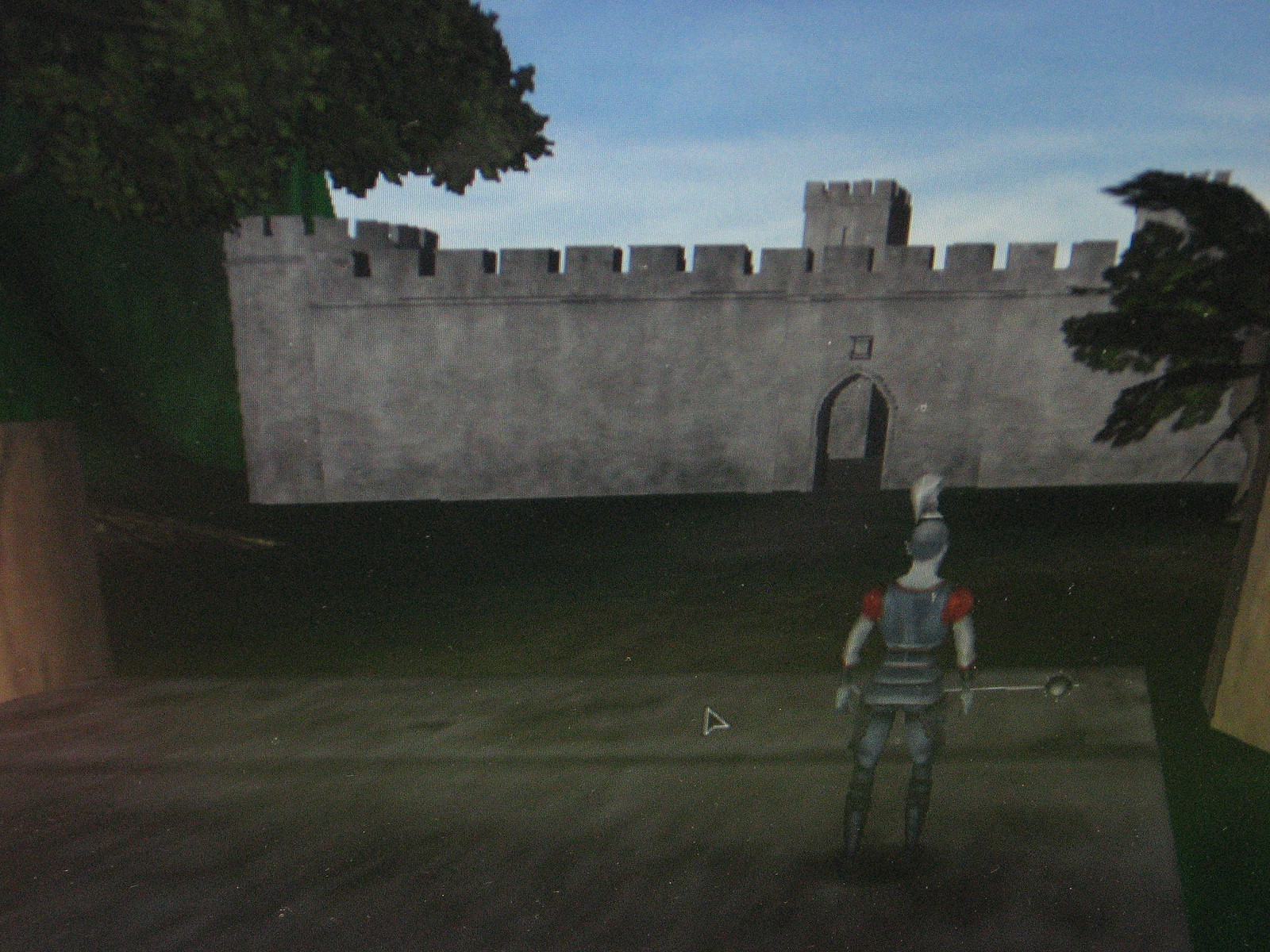In this highly detailed scene, reminiscent of a video game environment, we observe the fortified entrance to a medieval castle, encapsulated by formidable stone walls. The entrance itself is distinguished by an arched gateway, framed by meticulously placed stone blocks that merge seamlessly along the top of the wall. Dominating the backdrop, a towering stone structure looms, adding to the imposing presence of the castle.

Standing resolutely in front of the entrance, a solitary knight commands attention. Adorned in a gray tunic accentuated with black horizontal stripes or layered sections, he presents a formidable figure. His attire is further complemented by gray tights beneath leather chaps around his thighs, and a short-sleeved red shirt peeks out from under his tunic. His long blonde hair is neatly pulled into a ponytail atop his head, heightening his valiant appearance.

In his hands, the knight grips a formidable weapon—a polearm crowned with a spiked, ball-like head—emphasizing his readiness for battle. Surrounding the castle walls and extending into the foreground, we see massive tree trunks and towering trees, their natural grandeur juxtaposing the man-made strength of the stone fortress, creating a scene rich with medieval austerity and natural beauty.